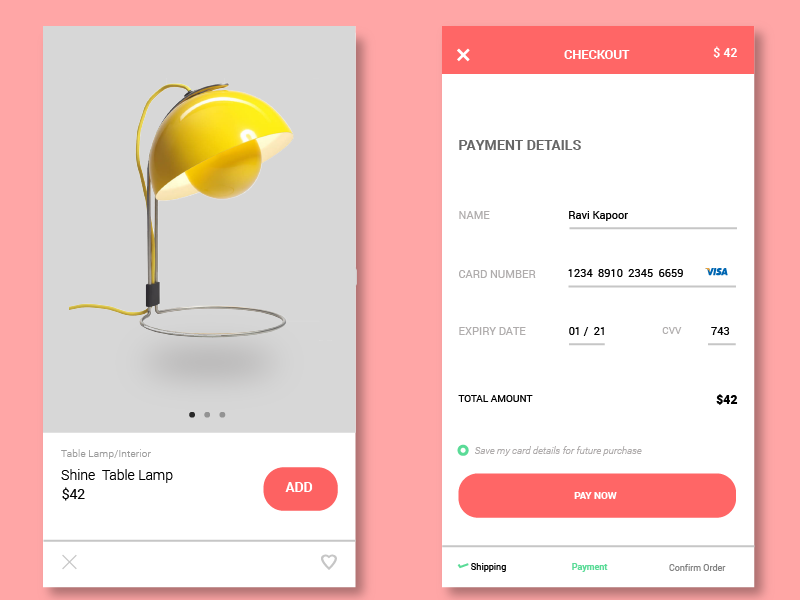The image is a composite screenshot featuring two distinct sections, set against a vibrant night pink background. 

**Left Section: Product Details**
- The left box showcases a sleek, modern table lamp. The lamp, with a gray background and a shade, features a vibrant yellow bulb. Its standard design includes a downward line leading to a circular base.
- Below the lamp image, there's a row consisting of a black dot followed by two gray dots.
- At the bottom, framed by a white border, the text on the left-hand side reads:
  - **"Table Lamp / Interior"** - Denoting the category.
  - Underneath, **"Shine Table Lamp"**
  - Price: **"$42"**
- To the right of the price, a prominent red bar displays the word **"Add"** in white text.
- A gray line separates the product details from other information.
- In the top-left corner, a gray "X" is visible, likely indicating a close or dismiss function.
- The bottom-right corner has a gray heart outline, possibly for favoriting or wishlisting the item.

**Right Section: Checkout Details**
- At the top of this section, a red bar spans across, featuring a white "X" on the left and the text **"Checkout"** in the center. On the right-hand side of the bar, the price **"$42"** is displayed in white.
- Below, the heading **"Payment Details"** is printed in black on a clean white background.
  - **"Name"** - In gray text, followed by **"Robbie Kapoor"** in the black text to the right.
  - **"Card Number"** - Gray text with the input **"1-2-3-4-8-9-1-0-2-3-4-5 6-6-5-9"** and a **"Visa"** indication in blue.
  - **"Expiry Date"** - Gray text with **"0-1-2-1"** next to it in black and underlined.
  - **"CVV"** - Gray text with **"7-4-3"** to the right in black.
    - **"Total Amount"** - Bold black text with the total **"$42"** to the right.
- Underneath, there's a gray circle with a white circle inside it, followed by **"Save my card details for future purchases"** in gray.
- A white bar for **"Pay Now"** in white text below the total amount.
- At the bottom, the words:
  - **"Shipping"** - in black.
  - **"Payment"** - in green.
  - **"Confirm Order"** - in gray text on the right.

This detailed screenshot creatively merges product selection and checkout processes, streamlined into a cohesive, visually striking presentation on a pink-hued backdrop.